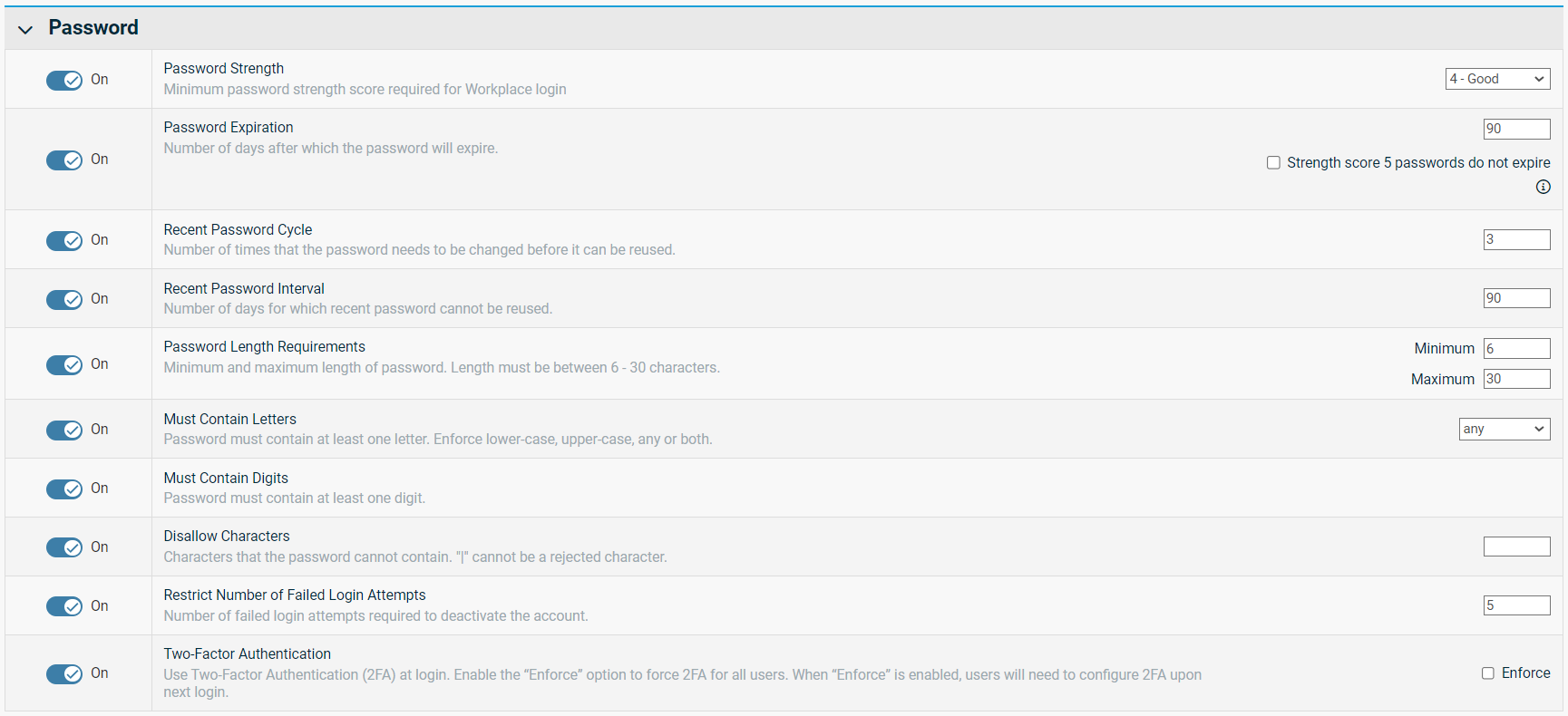Screenshot of Password Settings Interface:

The image displays a user interface for configuring password settings, which appears to be from a workplace-related system or application, though no specific website URL or name is visible. The background features a grayish hue, with predominantly black and light gray fonts used to differentiate titles from descriptions.

In the top left corner, the word "Password" is prominently displayed in bold black font. Adjacent to this, a small downward-pointing arrow is visible, likely serving to expand or collapse the section.

Below the title, various toggle buttons are visible, and all are currently toggled on. These toggles correspond to multiple sections within the password category, each governing different security parameters. The sections include:

1. **Password Strength**: Enforces criteria to ensure passwords are robust.
2. **Password Expiration**: Sets the timeframe for how long a password remains valid.
3. **Recent Password Cycle**: Governs the reuse of recent passwords.
4. **Recent Password Interval**: Defines the waiting period before a password can be reused.
5. **Password Length Requirements**: Specifies minimum and maximum password lengths.
6. **Must Contain Letters**: Requires passwords to include alphabetic characters.
7. **Must Contain Digits**: Requires passwords to include numeric characters.
8. **Disallow Characters**: Sets limitations on specific characters that cannot be used in passwords.
9. **Restrict Number of Failed Login Attempts**: Limits the number of unsuccessful login attempts.
10. **Two-Factor Authentication**: Adds an extra layer of security by requiring a second form of identification. 

Each section provides options to set various parameters, ensuring comprehensive security customization for the users' passwords.